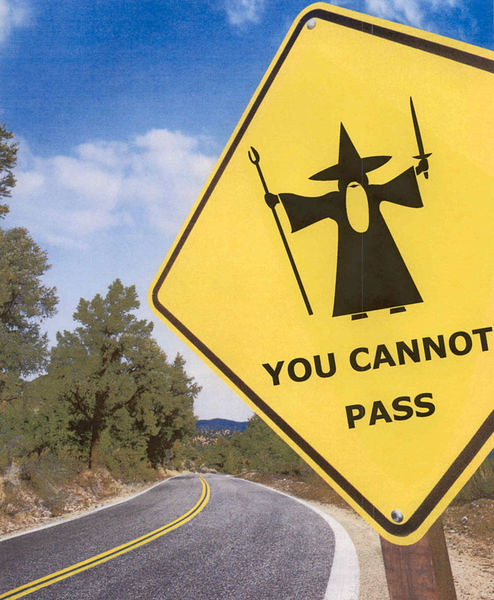The image depicts a yellow, diamond-shaped sign featuring a detailed illustration of a wizard. The wizard is brandishing a staff in his right hand and a sword in his left. Clever use of negative space in the wizard's torso gives the impression of a long flowing beard. The sign prominently displays the warning text "You Shall Not Pass." In the background, a road stretches out beneath a vibrant blue sky dotted with fluffy clouds. On the left side of the road, there is a cluster of lush green trees, while the right side shows patches of brown dirt interspersed with green shrubs.